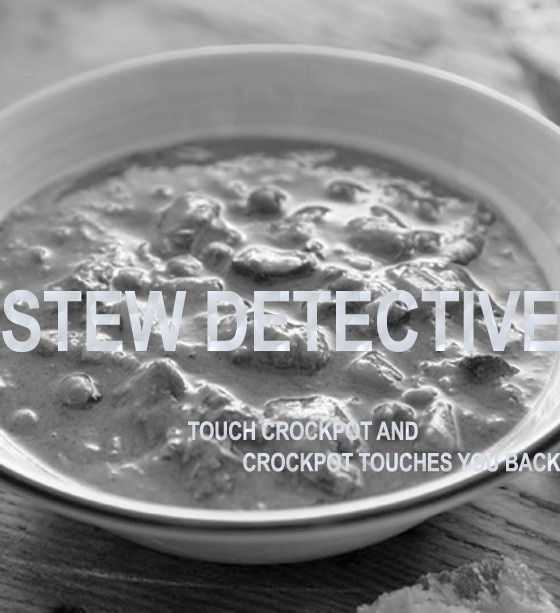This black and white image showcases a square photo of a large, white, round bowl filled with chunky stew, which likely consists of beef and vegetables. The bowl is centrally positioned, with both its left and right sides cut off by the image's borders, emphasizing its prominence. It rests on a wooden table, evident from the visible grain patterns beneath it. The background at the top is a blurred gradient of gray shades, which contrasts with the sharper texture of the table below. In the middle of the image, large white all-caps text reads "STEW DETECTIVE," and just below that, in smaller all-caps letters, there’s the phrase, "TOUCH CROCKPOT AND CROCKPOT TOUCHES YOU BACK." In the bottom-right corner, there's an unidentifiable object with a ragged edge. The overall composition and color scheme, featuring white, black, and various shades of gray, suggest the image could be from a kitchen, a restaurant, or possibly a page from a cookbook.